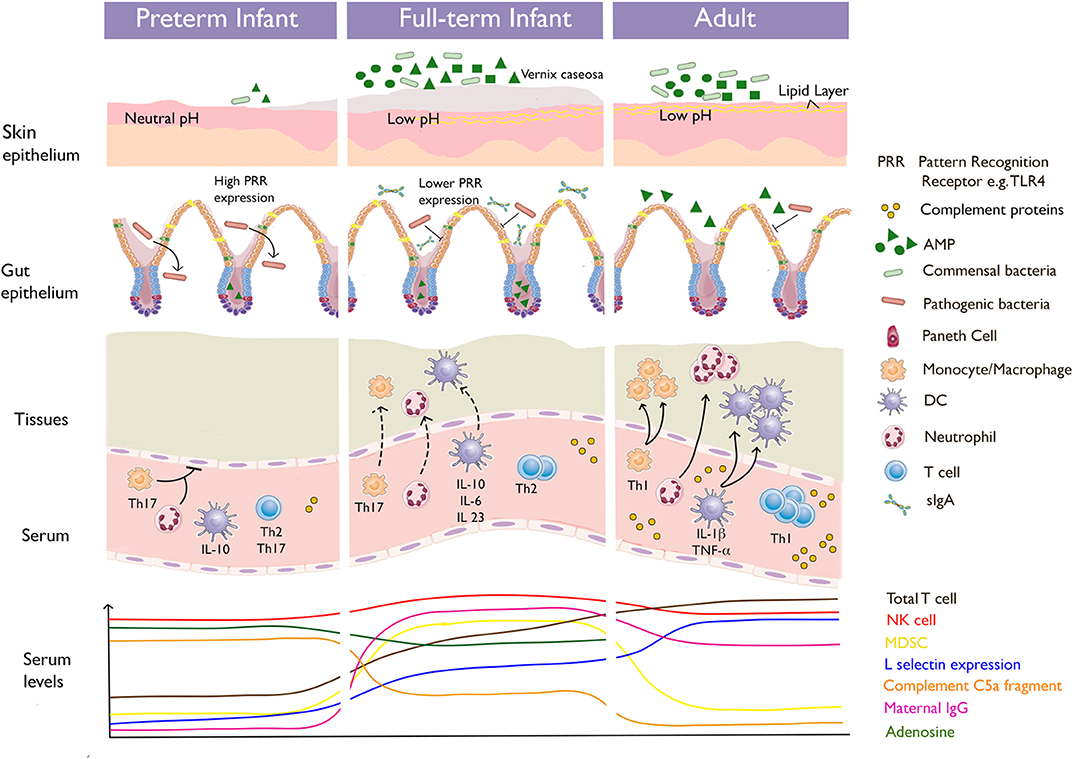This detailed scientific illustration, likely derived from a medical textbook or similar educational material, compares biological characteristics across three developmental stages: preterm infant, full-term infant, and adult. The top of the chart features lavender banners with white font labeling these stages. The diagram is divided into three columns, each representing one of the developmental stages, and five rows showing comparisons across different biological parameters: skin epithelium, gut epithelium, tissue composition, serum, and serum levels.

Each row includes detailed illustrations, showing layers of skin and gut epithelium, histological tissue differences, and various serum components. The illustrations are rich with colored lines and shapes—such as circles, squares, and triangles—each representing specific cells like T cells, neutrophils, and other biological entities such as complement proteins, AMP, commensal bacteria, and pathogenic bacteria. A comprehensive key on the right side of the image deciphers these symbols and shapes.

Furthermore, below the tissue and serum rows, a complex chart depicts serum levels with color-coded lines (red, green, purple, blue), indicating the concentration of various immunological components across different age groups. The legend assists in interpreting these levels, explaining terms like total C cell, NK cell, MDSC, L cyclone expression, complement C5A fragment, and maternal IgG. Overall, this diagram provides a thorough, technical visualization of developmental biology suitable for scholarly or educational use.